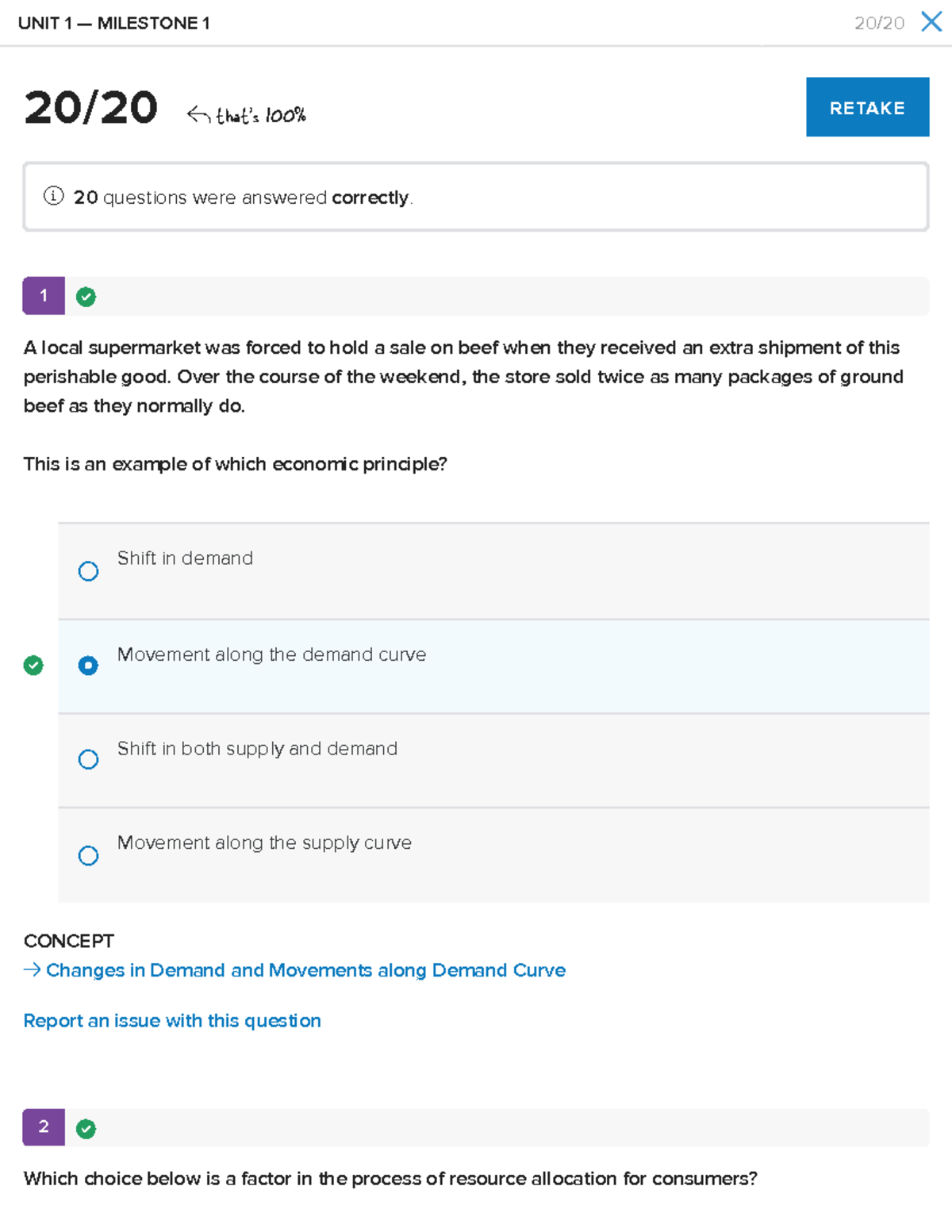The image displays a detailed assessment summary with various elements. At the top left, it reads "Unit 1 - Milestone," and on the top right, it displays "2020" alongside a blue 'X'. Below this header, a gray line separates the contents, followed by "2020" and "20/20." A black arrow points to a note stating "100%," indicating a perfect score. On the right, there is a blue button with white text labeled "Retake."

Further down, within a horizontally elongated rectangle, there is a white information icon inside a blue circle, stating, "20 questions were answered correctly." Adjacent to this, a purple box with a white number "1" is visible. The next section contains a field with a green circle and a white checkmark, presenting a scenario: "A local supermarket was forced to hold a sale on beef when they received an extra shipment of this perishable good. Over the course of the weekend, the store sold twice as many packages of ground beef as they normally do. This is an example of which economic principle?"

Following the scenario, there is a multiple-choice list with options, each preceded by a circle:
1. Shift in demand
2. Movement along the demand curve (checked)
3. Shift in both supply and demand
4. Movement along the supply curve

The option "Movement along the demand curve" is selected and highlighted with a green circle containing a white checkmark.